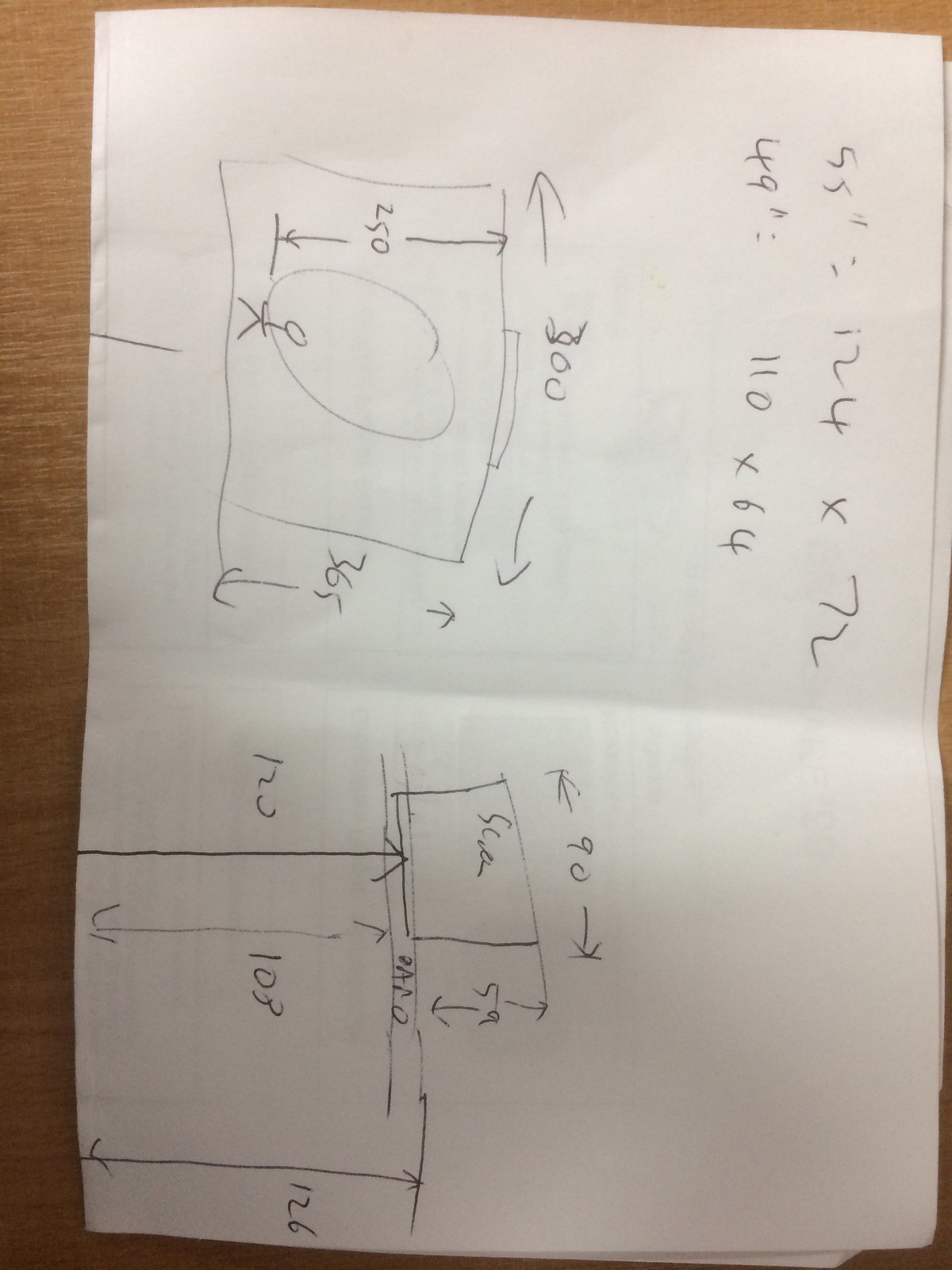This photograph captures a brown wooden table as its focal background. Centered on the table is a piece of white paper folded in half, lying on its side. The paper features multiple lines of handwritten text and illustrations. 

At the top of the page, there is an array of digits and mathematical symbols. The first line reads "55..12 x 4, 7, 2". Below this, a second line appears, stating "49..11 x 6, 4". Further down, the paper showcases a square with a circle inscribed within it. Inside the circle, there is a stick figure drawn. Surrounding this stick figure and the geometric shapes are various numerical annotations and directional arrows.

To the left side of the circle, two arrows point to a number "250". Above the circle, another set of arrows points to "300". To the right of this section, more arrows indicate "365". Adjacent to these illustrations is a noticeable fold in the paper, beside which there is a "90" marked with arrows.

Further, there is a box containing indeterminate text, flanked by arrows indicating "59". Below this, several lines and arrows lead to another box that says "12 C", accompanied by additional notations: "103" and "126" with corresponding arrows.

The combination of numbers, symbols, and arrows suggests that the paper might contain calculations, possibly a diagram or a schematic representation, or a layout plan.